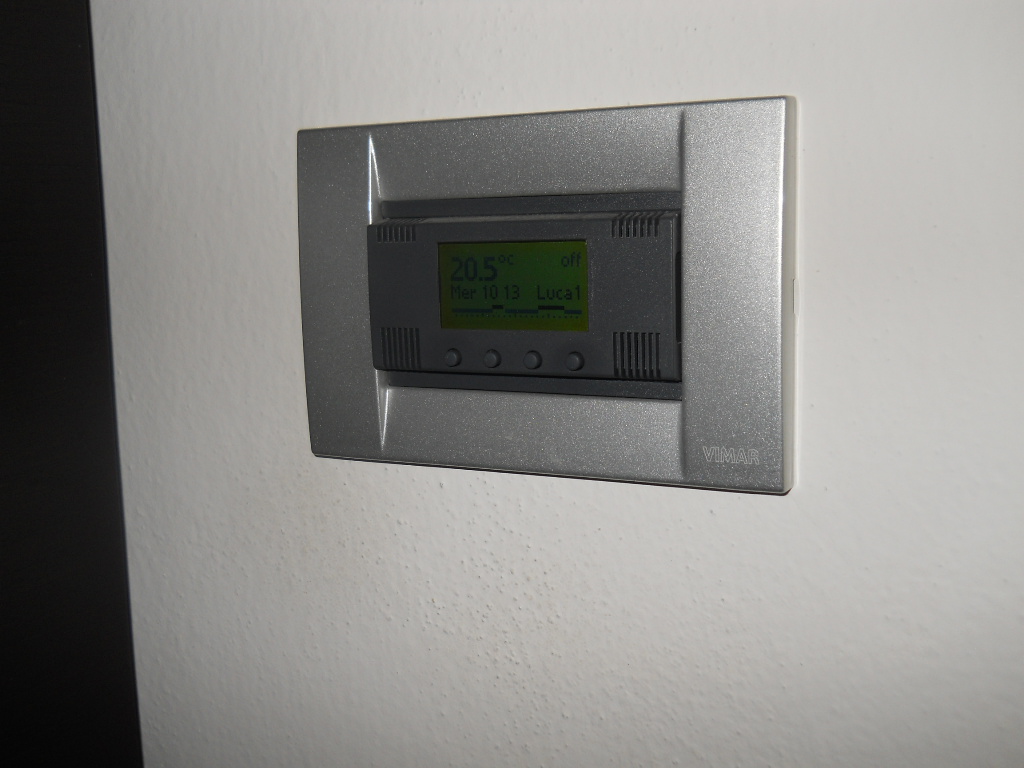The image depicts an interior wall of a house or building, featuring an off-white, slightly textured surface reminiscent of goosebumps. This wall exhibits signs of age and use, giving it a well-lived-in appearance. On the left side of the photo, a dark brownish-black stripe extends vertically, occupying about 10% of the image's width. The stripe is slightly narrower at the top than at the bottom.

Dominating the right section of the image is a silver instrumentation panel mounted on the off-white wall. The panel, identified by the white-outlined lettering "VIMAR" at the bottom corner, is framed by a silver bezel. Central to the panel is a gray rectangle with four buttons positioned at the bottom. This rectangle features decorative fins on both the top and bottom, arranged in sets of six to eight, with the bottom fins being slightly taller.

The centerpiece of the panel is a green LED screen displaying information, likely related to an HVAC system. The screen reads "20.5" in large digits, with the word "OFF" in smaller letters beside it. Beneath this, additional writing, possibly "March 1013 LUCA 1," is partially visible but not clearly legible.